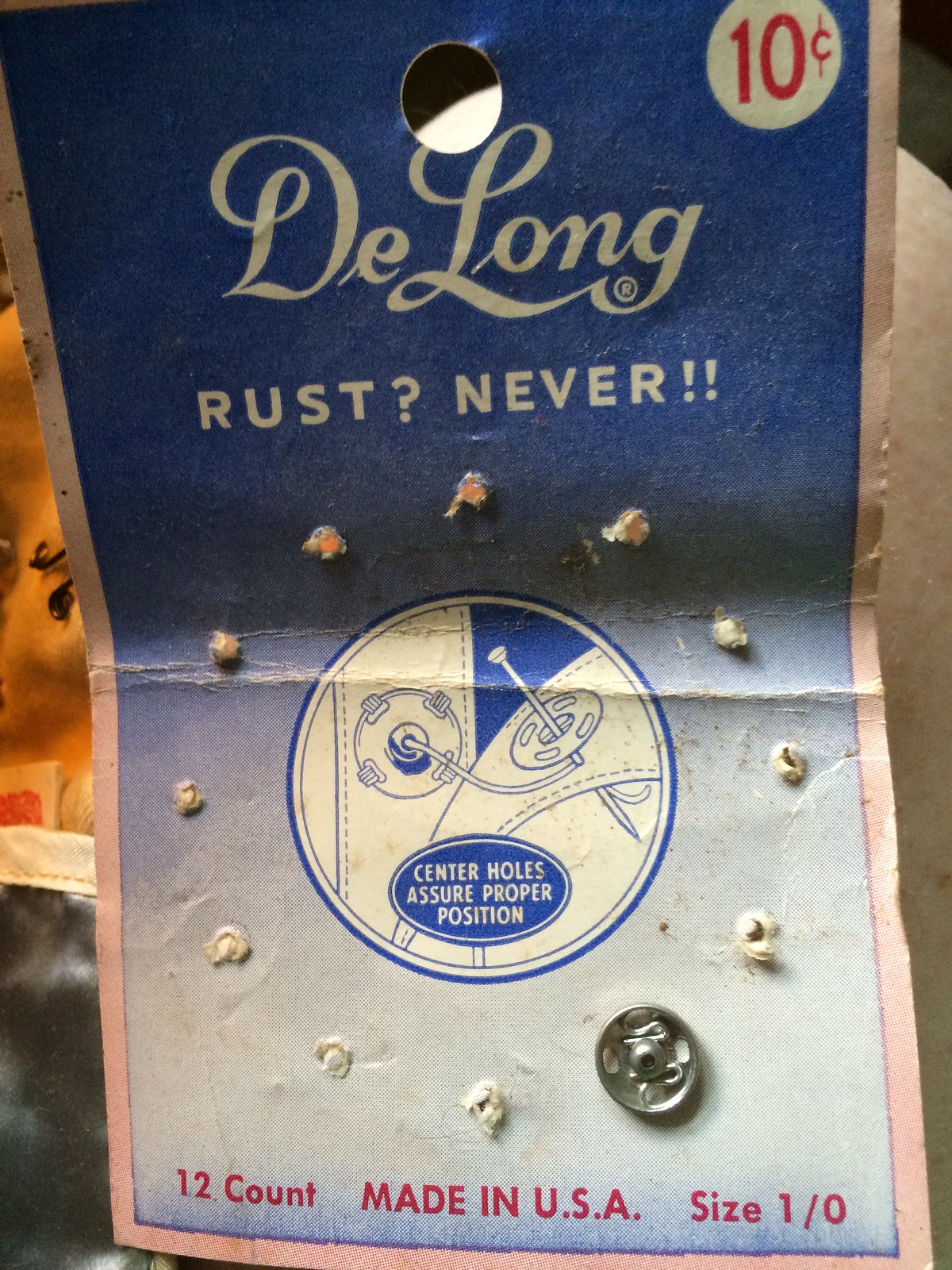The image depicts a vintage packaging from the 1950s or 1960s, originally holding 12 silver buttons, with only one remaining. The packaging, likely designed for sewing enthusiasts, features a blue booklet with intricate white script that reads "DeLong – Rust? Never!" emphasizing the rust-resistant quality of the buttons. At the bottom of the packaging, it states "12 count, made in the USA, size 1/0" in red text. Additionally, there's a detailed illustration in the center showing a button being sewn, suggesting its use for replacing or adding buttons to clothing. The price, remarkably set at just 10 cents, is prominently displayed in the top corner, indicative of its age and affordability at the time. The frayed paper and sparse button holes poignantly highlight the item's extensive use over the years.